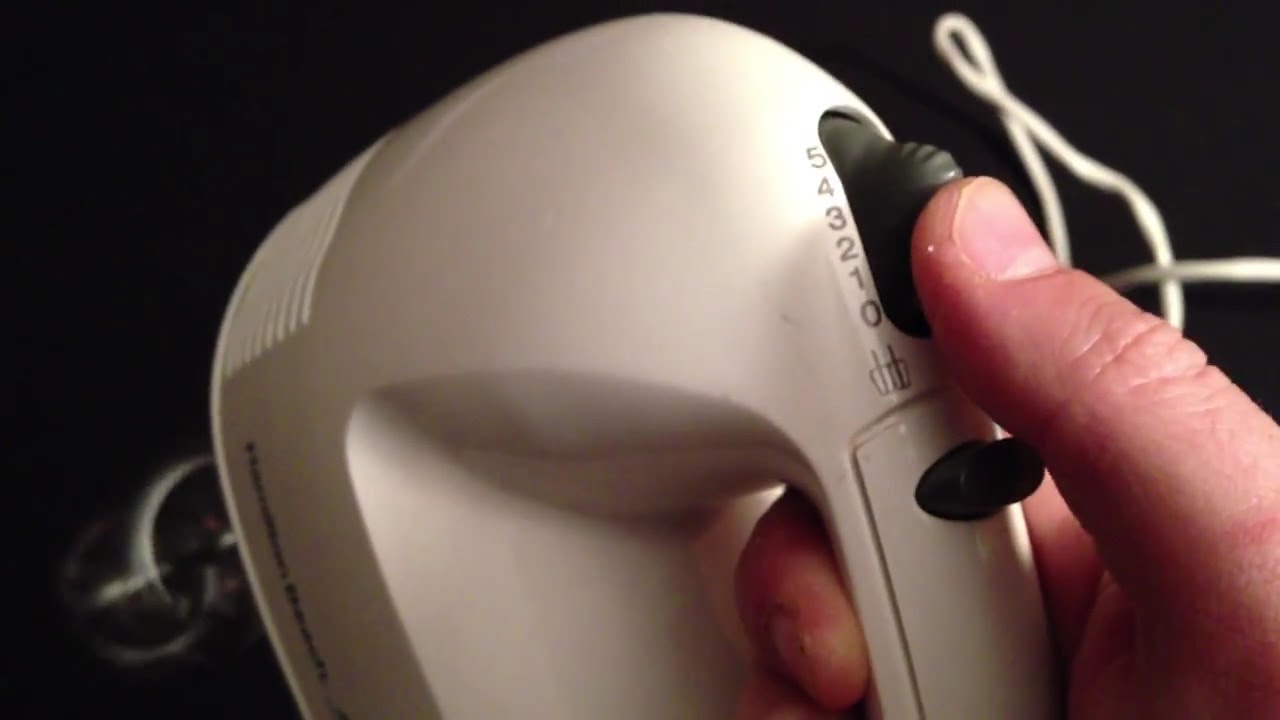This is an extreme close-up image of a handheld electric mixer, predominantly white in color. The focus is primarily on the control section of the mixer, where a light-skinned person's thumb is engaging a gray switch that adjusts the speed settings, which range from 0 to 5, displayed in lighter black numerals. Another button located below the switch functions to release the whisk attachment. The person’s hand is firmly gripping the handle, with additional fingers visible beneath it, reflecting a secure hold. The mixer bears the brand name "Hamilton Beach," although the text is slightly out of focus. The mixer’s base transitions into a silver bar that supports the whisk attachment, seen in a circular motion at the bottom left of the image. In the upper right of the frame, the mixer’s white cord is faintly visible but out of focus, set against a solid black background.